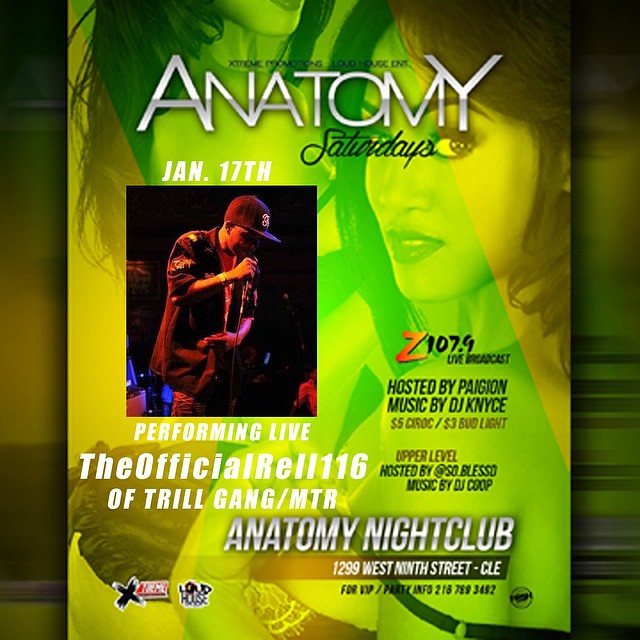The image is an advertisement poster for "Anatomy Saturdays," prominently displayed at the top in large white and silver letters. The background features a sultry, makeup-clad woman, her image filtered with green and yellow hues. Another similar image shows two attractive women, their faces and part of their bodies visible, enhanced by an orange filter. On the left side, there's a smaller picture of a man, who appears to be a rapper or DJ, performing with a microphone in his right hand, wearing a dark cap, hoodie, jeans, and a black shirt. The text includes the event date, January 17th, followed by "Performing Live: The Official REL 116 of Trill Gang/MTR." Sponsor logos line the bottom of the poster. On the right, it notes a Z107.9 live broadcast hosted by Pagion, featuring music by DJ Nice, with $5 Ciroc and $3 Bud Light on the upper level, the latter hosted by SO Blessed with music by DJ Coop. Contact information for VIP and party inquiries is provided, listing Anatomy Nightclub at 1299 West Ninth Street, with a phone number: 216-789-3452.